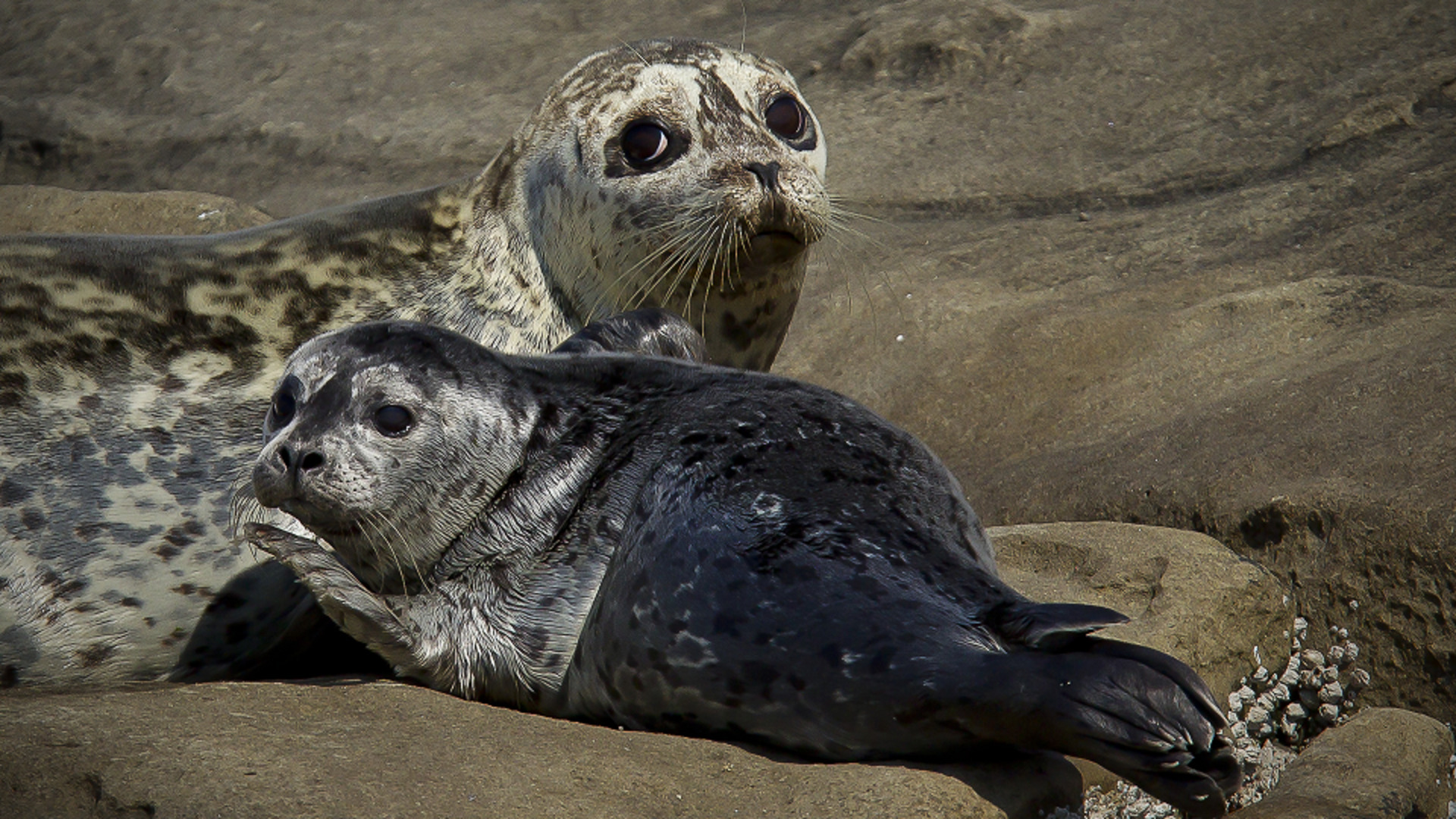A photograph showcases a pair of seals lying on a sandy-colored, rocky surface. In the foreground, a baby seal with a gray coat on its top half and black on the bottom is prominently visible. The small seal's left flipper is raised towards the camera, exposing its large, dark eyes that convey a sense of worry or fear. Behind this baby seal, a much larger seal, presumably the mother, can be seen. This adult seal features a white coat adorned with black designs and dots, and it observes the scene with a suspicious expression. Both seals have long, whitish whiskers that stand out against their contrasting fur. The different rocks around them vary in color, ranging from tan to darker browns, with some white shells growing on a nearby rock by the baby seal's foot. Despite the numerous rocks, there's no visible water in the scene.